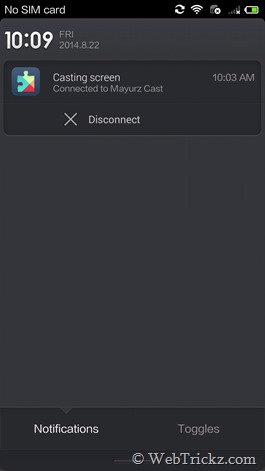The image displays a phone screen with a predominantly black background and white or light gray text. In the upper left corner, the status bar reads "No SIM card" and contains icons including a circular two-arrow symbol, a fully filled Wi-Fi icon, an obscured icon, and a cellular service icon marked with an 'X.' The battery icon indicates approximately 50% charge with a green color. The time shown is 10:09 on Friday, August 22, 2014.

Central to the screen is a notification featuring a multicolored puzzle piece icon. The icon transitions from green (left) to yellow (top) to orange (right) and finally to a small red triangle at the bottom. The text below this icon states, "Casting screen connected to Mayor's Cast at 10:03 a.m." with an 'X' icon provided to disconnect the casting.

Directly below this is a small downward-facing caret, indicating further notifications available below. The screen shows that it is in the notifications context. To the right, there's an option to switch to toggles. The very bottom of the screen is marked with "Copyright webtrickz.com," with ‘tricks’ uniquely spelled as 'T-R-I-C-K-Z.'

Overall, the screen appears relatively uncluttered, primarily focused on the detailed status and notifications.